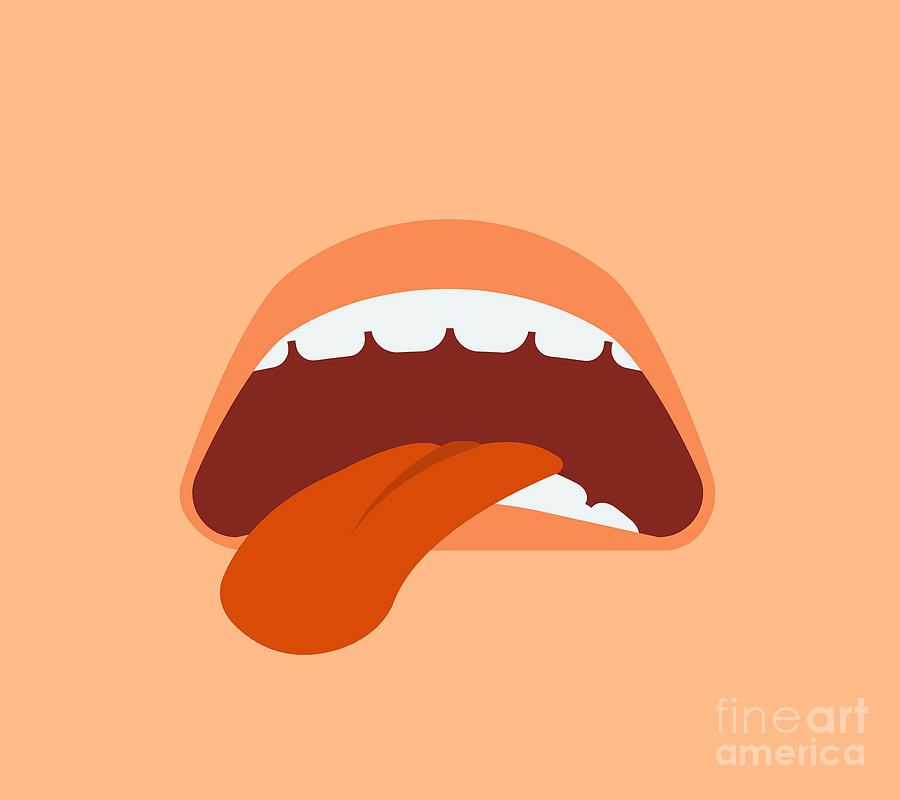This digital artwork, titled "Fine Art America" as indicated by the watermark in the bottom right corner, features a stylized, abstract depiction of an open mouth with its tongue sticking out. The overall background is a light orangey beige, providing a neutral backdrop that complements the vibrant elements of the mouth. The lips are a contrasting lighter and darker orange, highlighting their shape, while the teeth are prominently white and straight. Within the open mouth, a dark burgundy hue serves as the backdrop, showcasing a bright red-orange tongue that protrudes to the right. The simplistic yet striking design of the piece is reminiscent of modern pop art, evoking similarities to the iconic Rolling Stones logo. The entire composition is encapsulated in a rectangular frame, emphasizing its minimalist and bold visual style. The expression conveyed by the mouth, with its slight frown and protruding tongue, suggests a sense of displeasure or distaste, adding a layer of emotional depth to the artwork.